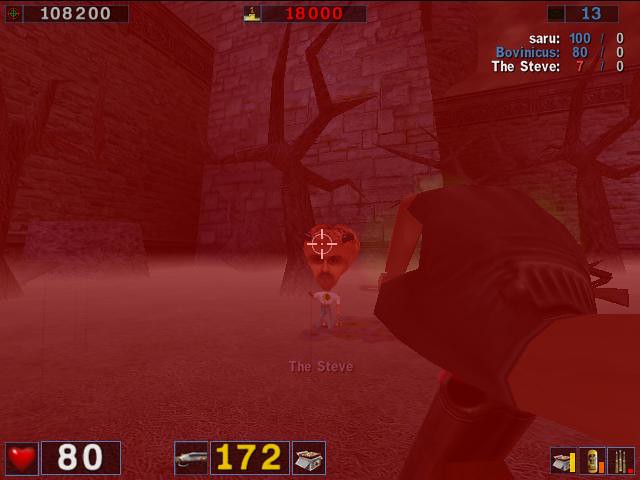Screenshot from a video game: The image features the player character reloading a shotgun, with the crosshair targeting an oddly proportioned character named "The Steve." This character has an enormous head paired with a minuscule body, dressed in a white shirt and blue pants. "The Steve" is positioned with one arm raised while the other hangs limply.

The user interface of the game displays several elements: 
- At the top of the screen, the numbers "18,000" and "108,200" are shown in the center and top left, respectively.
- The top right corner includes the number "13" and further details: "Saru, 100 out of 0," "Bovenikas, 80 out of 0," and "The Steve, 7 out of 0."
- A health gauge at the bottom reads "80," accompanied by a 3D heart icon.
- Adjacent to this, yellow text displays "172," flanked by a shotgun icon on the left and a box of shells on the right.
- Three additional icons are visible in the bottom right corner.

The background depicts cinderblock walls and dead trees, all rendered in 3D graphics, characteristic of video game environments.